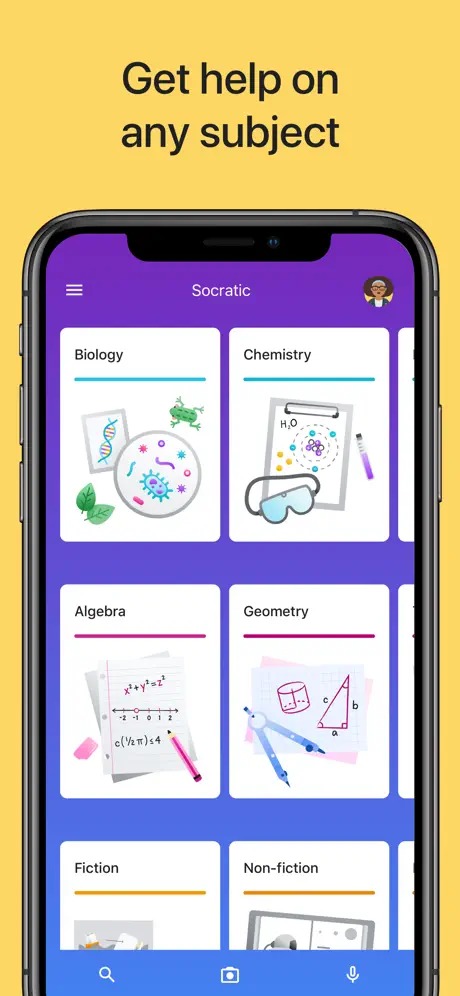**Advertisement Caption for Socratic App or Service**

This advertisement features a vibrant promotion for the Socratic app or service, set against a striking yellow background. At the top, in bold black text, the tagline reads, "Get help on any subject." 

Central to the ad is an image of a sleek, black iPhone displaying the Socratic app interface. The smartphone screen showcases a dynamic bluish-purple background with the Socratic logo at the top, accompanied by a hamburger menu on the left. There is a circular user profile image, likely a photograph or a caricature of the user, providing a personalized touch to the user interface.

Below the profile section, the interface displays a series of subject area tiles arranged in rows, although only six are partially visible. These tiles have cartoonish images representing various subjects. For example, the biology tile features illustrations such as DNA, a frog, a cell schematic, and leaves. The visible subject areas include Biology, Chemistry, Algebra, Geometry, Fiction, and Nonfiction. Each row of tiles appears organized by themes: Physical Sciences, Mathematics, and Reading or English.

Distinctive colored bars separate the titles from the illustrations on each tile – turquoise for sciences, purple for math, and yellow for reading and English. This color-coding adds to the visual organization and user-friendly design of the app.

At the bottom of the screen, set against the blue background, are white icons for different functions: a magnifying glass for search, a suitcase (the purpose of which is not immediately clear), and a microphone.

This detailed and visually engaging ad compellingly communicates the versatility and comprehensiveness of the Socratic app, making it an appealing tool for students across various subjects.